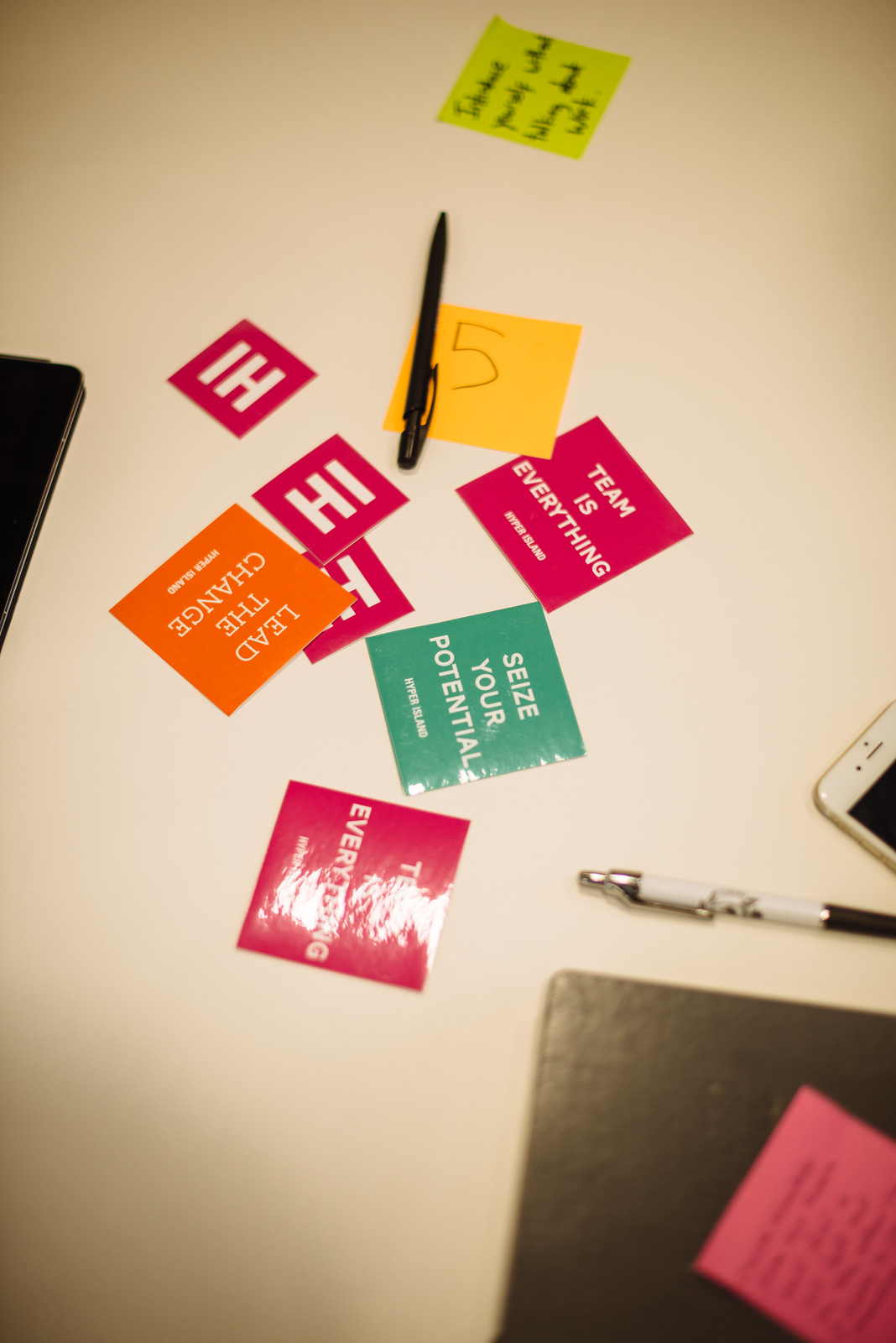This photograph captures a diverse array of items thoughtfully arranged on a pristine white desk, seemingly from someone's office. In the center, a colorful assortment of Post-it notes and cut-out pieces of paper lie prominently. A yellow sticky note, albeit blurred, stands out with bold black ink, while an orange sticky note features the number five. Other notes inspire with messages such as "Team is everything," "Seize your potential," "Lead the change," and several that simply say "Hi."

Two cell phones are visible, one placed to the left and the other to the right of the image. On the bottom right, there's a book or possibly a tablet face down, adorned with another sticky note. A pen is also present near the center, among the Post-its and paper pieces.

The color palette of the items includes striking hues of white, tan, black, pink, silver, red, orange, yellow, and light green, creating a visually engaging scene. The bright and clean background suggests an indoor setting, potentially in an office or a workspace. The precise arrangement of motivational notes and everyday office items gives the impression of a snapshot capturing the essence of productivity and inspiration.